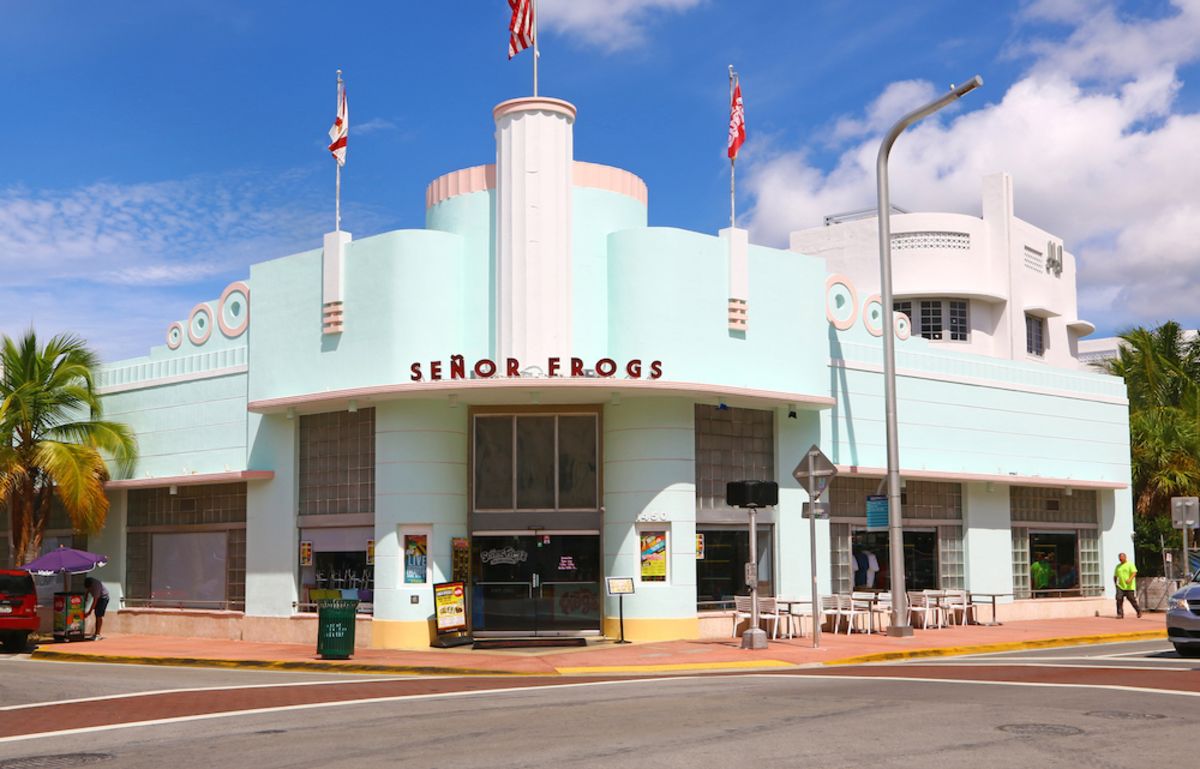The photograph depicts the vibrant exterior of the "Senior Frogs" building. Dominantly colored in a pale light blue, the structure features a round, cathedral-like top with a central American flag flanked by two additional flags. The front of the building is crowned with the establishment's name in bold red letters. Beige circles adorn both sides of the flags, adding to the architectural flair. The double glass doors serve as the main entrance, situated at the corner of the bustling street.

Outside, a lively scene unfolds with people strolling along the sidewalk, some dressed in bathing suits, suggesting a tropical locale. A sidewalk vendor with a distinctive purple umbrella stands to the left of the entrance, while white tables and chairs are arranged for outdoor dining. Various signs and advertisements are displayed near the front doors, providing information to passersby. The bustling street features vehicles, a green trash can, street lights, and lush palm trees under a beautiful blue sky with scattered white clouds, enhancing the overall lively atmosphere of this intriguing establishment.